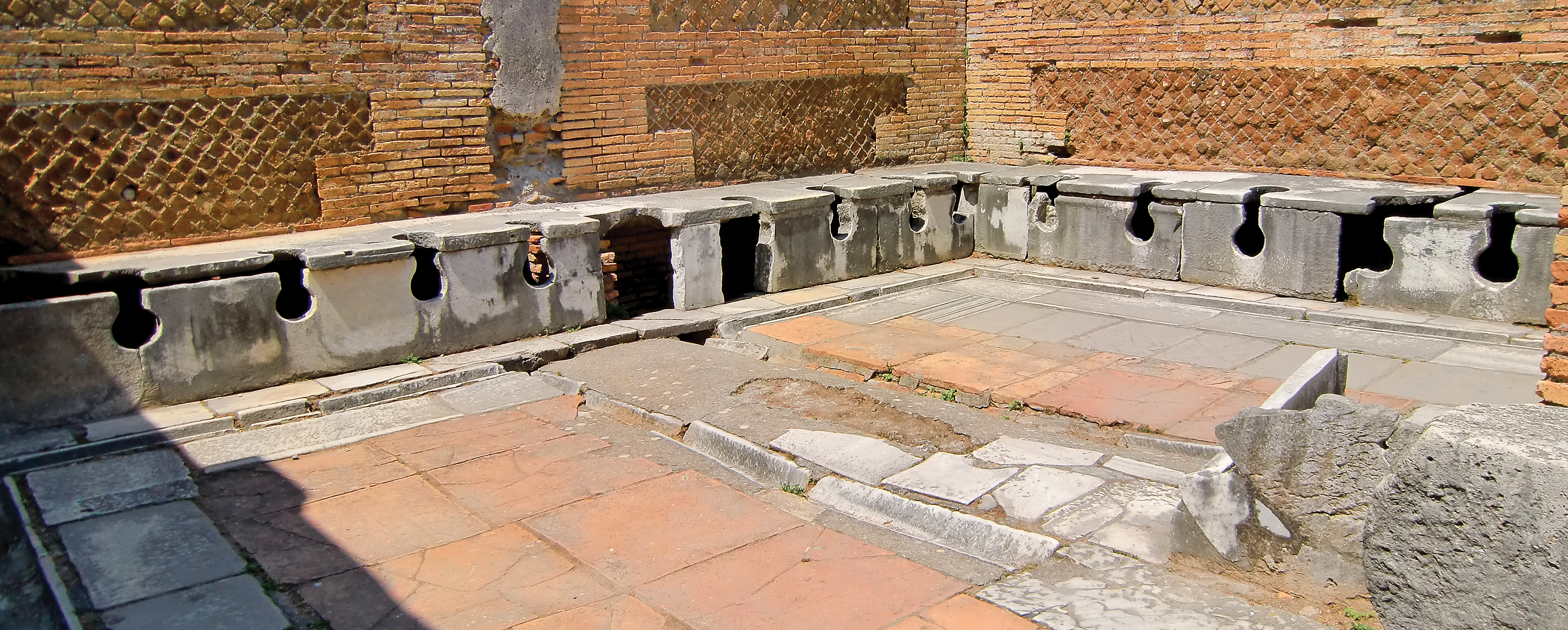This detailed photograph, taken in a bright outdoor setting with ample natural light, captures a well-lit landscape-oriented scene featuring dilapidated ruins. Dominating the upper third of the image is a reddish-brown brick wall arranged in a mix of diagonal and horizontal patterns, emphasizing its weathered and poorly maintained condition. Below this brick structure lies a concrete or gray bench that seamlessly transitions into a ground area paved with tiles of matching concrete gray and interspersed red shades. The overall scene exudes a sense of abandonment and disrepair, further accentuated by a patch of shade in the lower left-hand corner, suggesting the sun's position overhead. No identifiable objects, words, or numbers are present, maintaining a clear and unobstructed view of the stone surfaces and brick wall that make up the primary elements of the photograph.